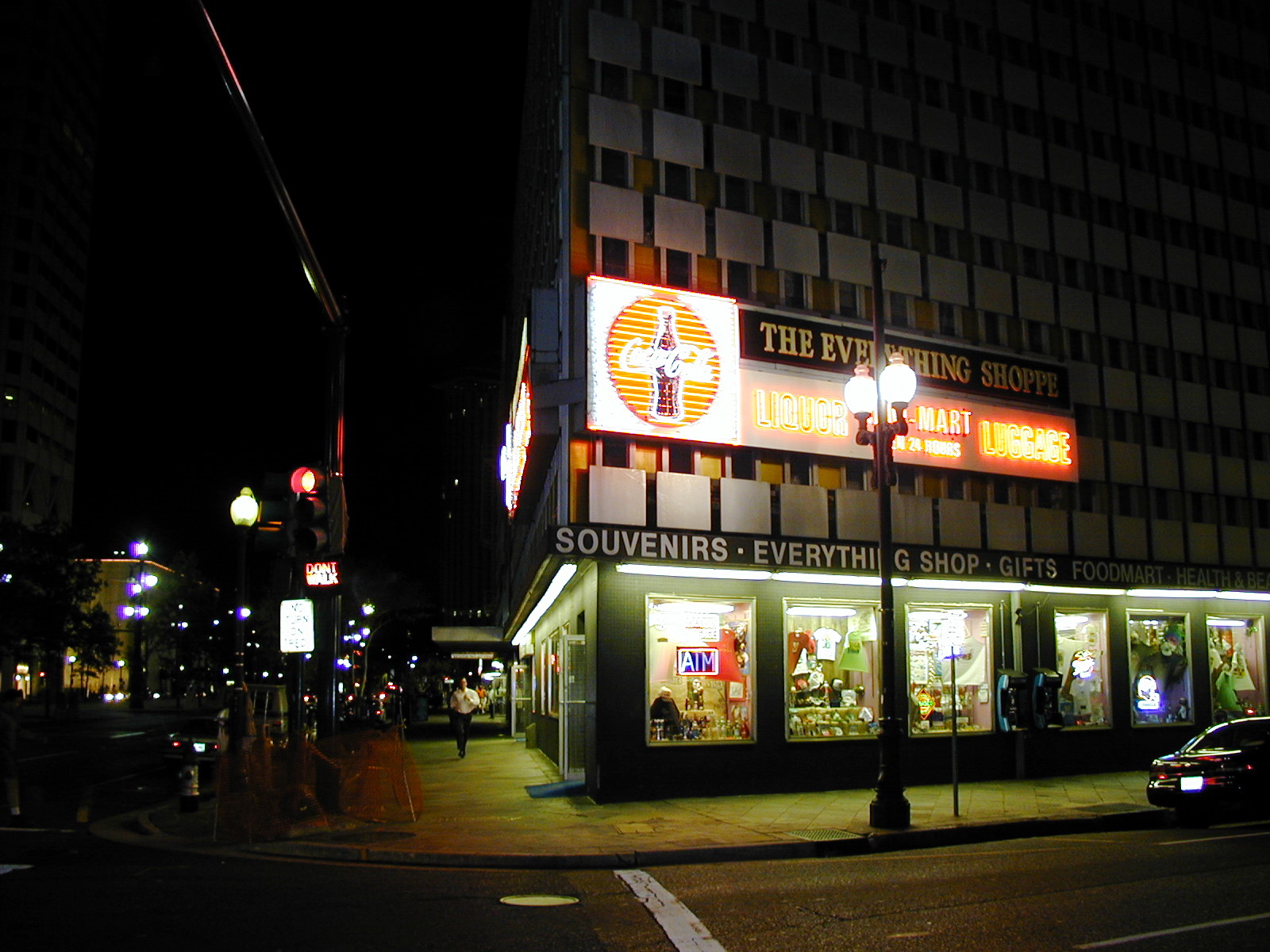A nighttime photograph captures a bustling urban street scene centered around a large, dimly-lit building adorned with a multitude of signs. The forefront banner, partially illuminated, reads, "Souvenirs, Everything Shop, Gifts, Food Mart, Health," with the remaining text obscured. Several windows dot the building’s facade, each casting a warm, inviting glow. One window reveals a person sitting amidst an array of indistinct objects, while another displays various clothing items. Above, another sign, partially lit, advertises "The Evening Shop, Liquor, Luggage," accompanied by an iconic Coca-Cola logo. The scene also features street lamps lighting the sidewalk, a car driving down the road, and a traffic light hovering above, completing this vibrant snapshot of urban nightlife.